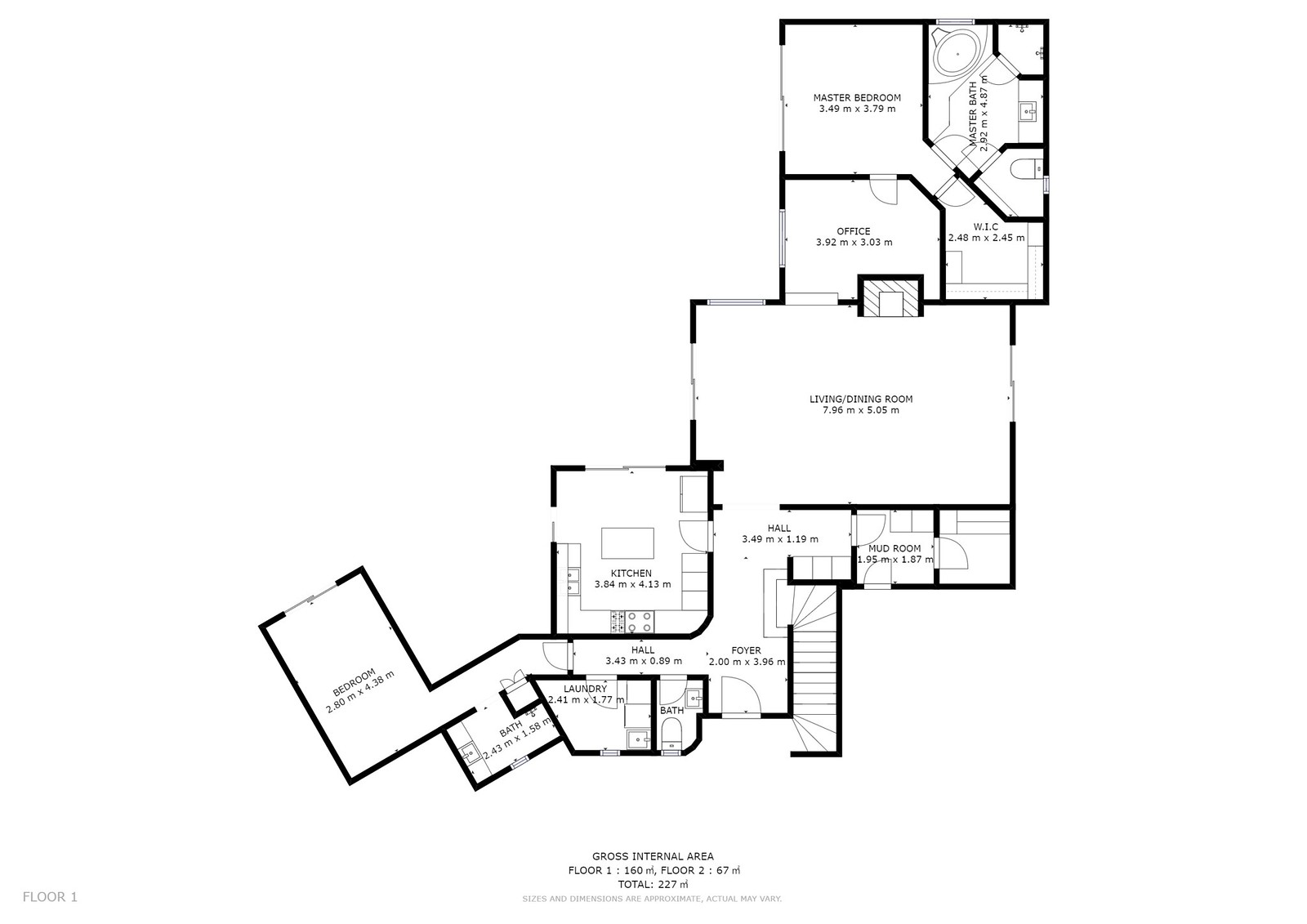A detailed architectural floor plan is depicted, presented on a white background with the layout details illustrated in black lines. At the bottom of the image, there is an annotation in black text that reads: "Gross Internal Area Floor 1, Floor 2, Total" accompanied by some numerical values too small to discern. In the lower left corner, the designation "Floor 1" is clearly marked.

Starting from the lower left corner of the blueprint, the layout begins with a bedroom. This bedroom opens into a hallway, which first leads to a bathroom. Continuing down the hallway, one encounters a laundry room followed by another bathroom situated opposite the laundry room. Still proceeding along the same hallway, you reach a kitchen, which is indicated as a square room. Adjacent to the kitchen, the hallway extends into a foyer, marking the formal end of the hallway. The foyer features stairs ascending to the upper floor and a front entrance door.

From the foyer, another hallway extends upwards, intersecting with the square kitchen. This further hallway passes by an additional bathroom and opens into a room without any labeled designation, leaving its purpose open to interpretation.